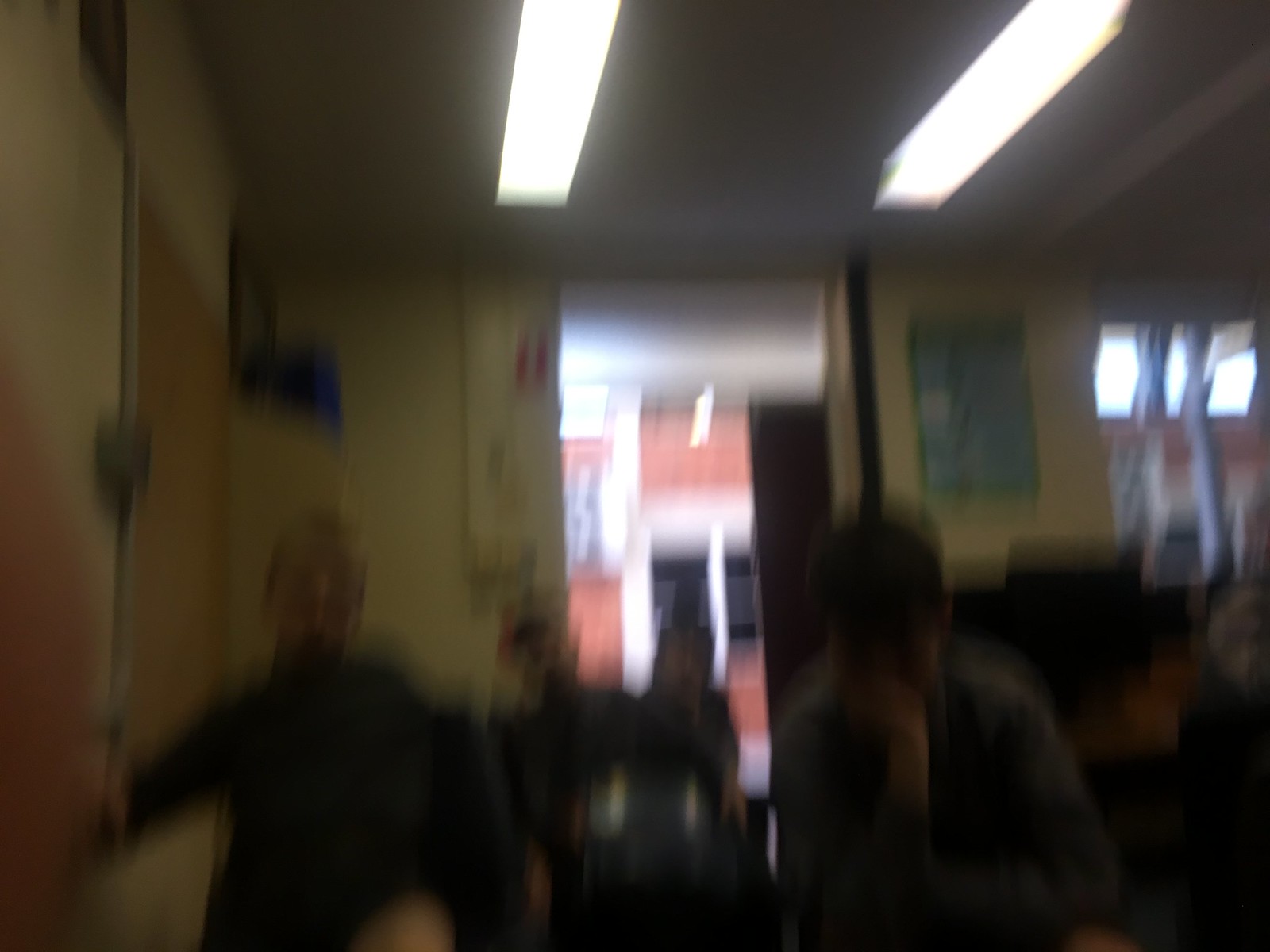The image depicts the blurry interior of a dimly lit room that has an off-yellowish-white or beige hue. Two long, bright white fluorescent lights illuminate the ceiling. Several people, likely children based on their height compared to a nearby door, are seen from the waist up, appearing to be standing, possibly in line or near a table or counter. To the room's far side, an open door reveals a brightly lit adjoining room with indistinct brown cabinetry. To the right of the door in the darker room, a green poster is visible, along with a cork board that has a metal trim. There's an outlet or a similar fixture near the cork board. Additionally, a blurred window can be seen at the top right corner of the image.